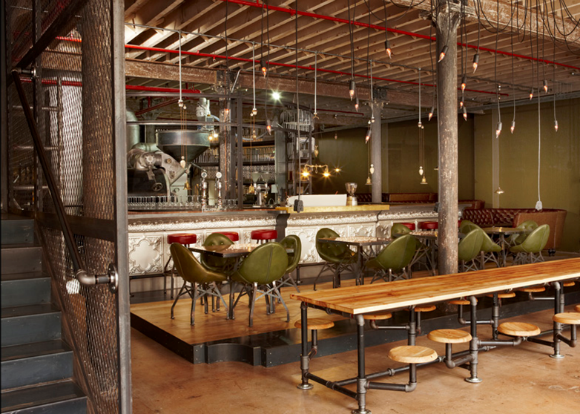The image depicts the interior of a modern, yet vintage-inspired establishment, possibly a restaurant or cafe. The space is characterized by an industrial design with exposed wood paneling on the ceiling and black cords suspending light bulbs. To the left, a dark grey, metal staircase ascends, contributing to the venue's rustic charm. Central to the room is a long brown wooden table with circular wooden stools attached. Surrounding this table is a wooden platform hosting three smaller tables, each accompanied by dark green leather chairs. In the background, there's an open area resembling a kitchen or workspace, furnished with greenish metallic machinery, typical bar glasses, and bottles. A white bar with red stools further enhances the retro yet contemporary atmosphere, while additional lounge seating with brown chairs offers varied seating options within this eclectic and thoughtfully designed space.